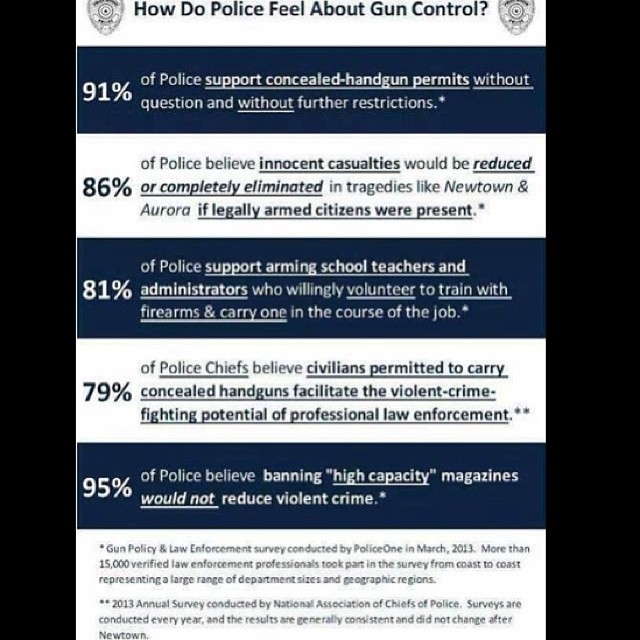This vertical rectangular poster features two prominent, dark black borders on either side, framing a series of alternating horizontal stripes in white and blue. At the top, in bold blue letters, it poses the question, "How do police feel about gun control?" The poster then provides detailed statistics on police perspectives regarding various gun control measures. It starts with 91% of police supporting concealed handgun permits without question or further restrictions, followed by 85% believing that innocent casualties could be reduced or eliminated in tragedies if legally armed citizens were present. Additionally, 81% of police support arming school teachers and administrators, while 79% of police chiefs believe that civilians permitted to carry concealed handguns enhance crime-fighting potential. Finally, at the bottom, it states that 95% of police believe banning high-capacity magazines would not reduce violent crime. The text alternates between blue and white, matching the corresponding background stripes, creating a visually organized and informative piece.